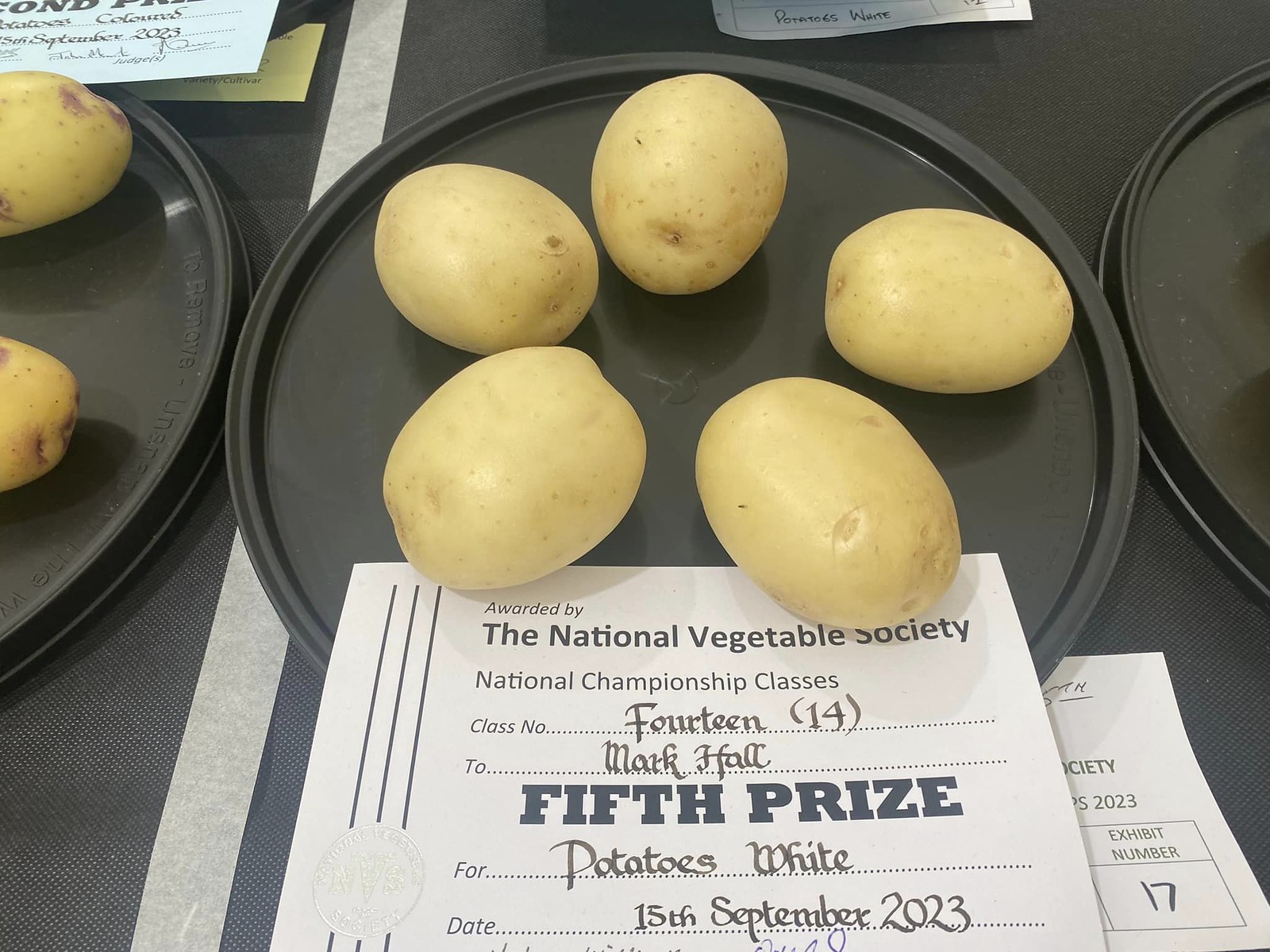The image features a black circular plate displaying five whole, perfectly round white potatoes. Positioned in front of the plate is a white card that reads, "Awarded by the National Vegetable Society, National Championship Classes, Class Number 14." The card indicates that the potatoes, which earned the fifth prize, were submitted by Mark Hall, with the award dated the 15th of September, 2023. Surrounding the central plate are partial views of additional dishes on either side, each containing cut-off halves of potatoes, emphasizing the presentation and competition of these prized vegetables.